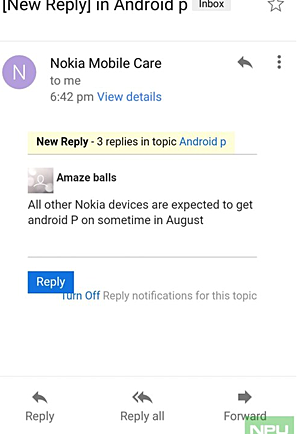The image depicts a notification screen from an Android Nokia mobile device, timestamped at 6:42 PM. At the top of the screen, there's a header stating "New Reply." Below this, a blue hyperlink labeled "View Details" is visible. On the left, there is a purple oval icon with a white capital "N", and to the upper right of this icon, it says "Inbox."

In the upper right corner, there are additional icons, including a left-pointing arrow, a star, and an ellipsis. At the bottom left of the screen, a tan rectangular box displays the message "New Reply." It indicates that there are three replies in the topic titled "Android P." The message within the box reads: "Amazeballs! All other Nokia devices are expected to get Android P sometime in August."

Beneath this message, there is a blue button labeled "Reply." Directly under the button, it says, "Turn off reply notifications for this topic." Following a blank space, there is a separating line, and below that, options to "Reply," "Reply All," and "Forward" are listed.